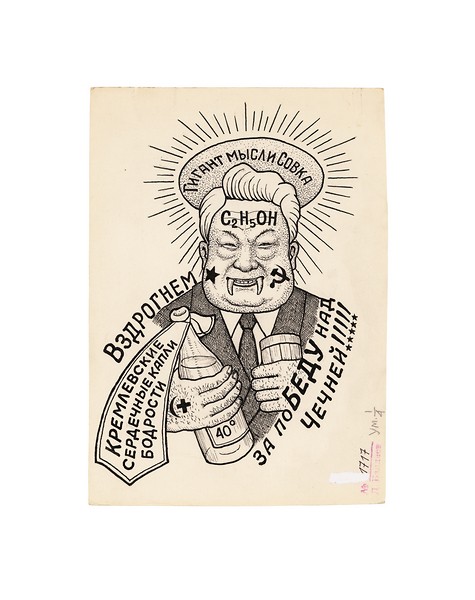Detailed Caption: 

The image is a detailed drawing on a tan piece of paper, featuring a man dressed in a gray business suit, complete with a gray tie and white shirt. The man has a chubby face, slicked-back hair, and a distinctive set of fangs protruding from his mouth. His eyes are squinting, giving him a somewhat menacing expression. Inscribed on his forehead is the chemical formula "C2H5OH," which denotes ethanol. 

On his cheeks, two notable symbols add to his ominous appearance: a black star on one cheek and the communist hammer and sickle on the other. The man holds a bottle bearing a white banner with text written in a foreign language in one hand, and a glass in the other hand, presumably containing a drink. Surrounding his head is a halo radiating light, which is adorned with additional foreign language text, enhancing the mystique of the image.